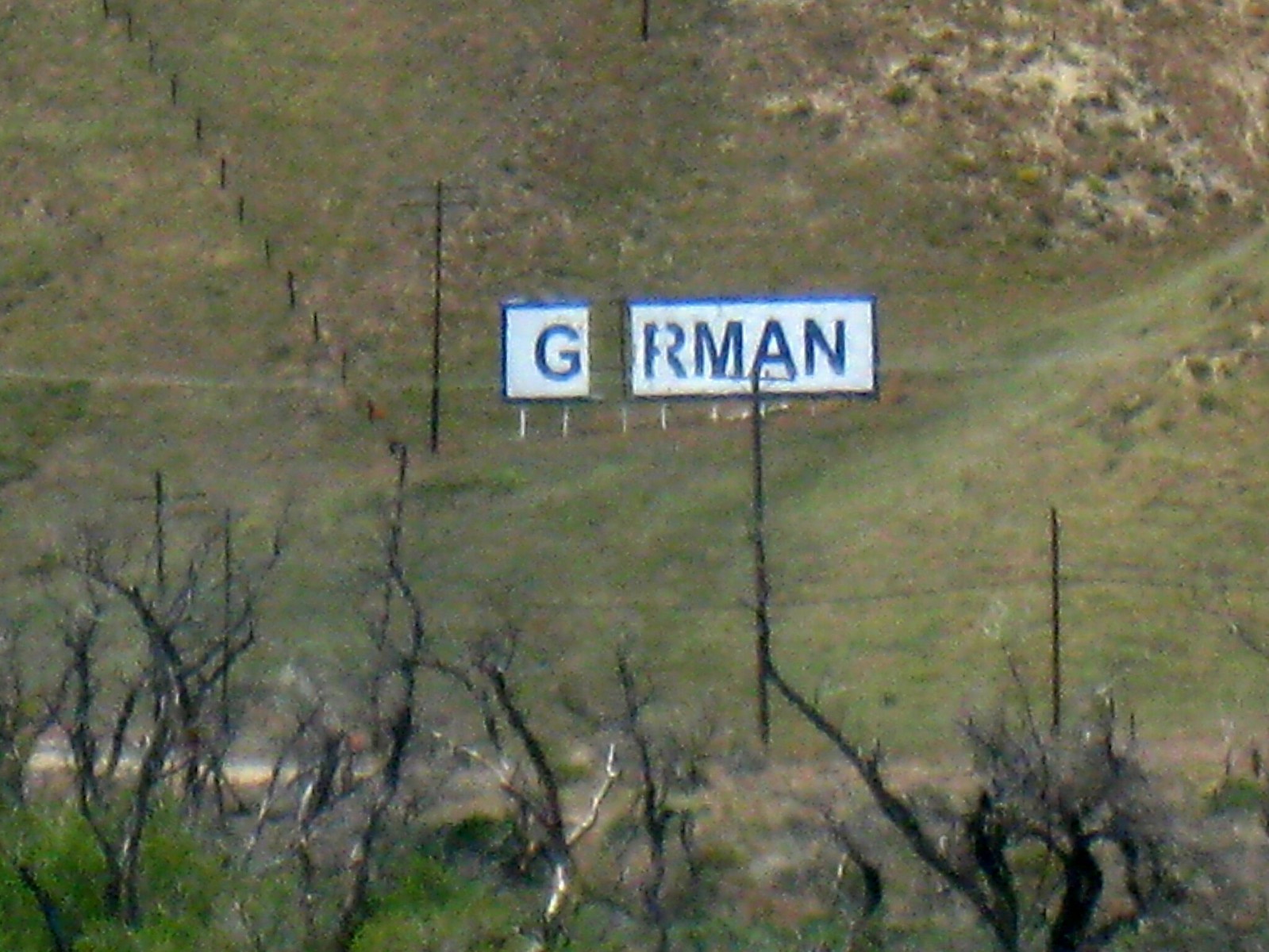The photograph captures a white billboard with blue text and a blue border, situated far out in rolling hills. The text on the sign is partially obstructed, reading "G R-M-A-N," with the letter between G and R missing, suggesting it might have originally spelled "German." This gap in the lettering reveals the background through the sign. Adjacent to the billboard, there are electrical poles, telegraph poles, and some fencing. The billboard is carefully positioned on a steep section of the hill, ensuring it is level. In the foreground, there are branches, trees, and vegetation. The hill itself is mostly covered in green grass, with soil and stones visible further up. The scene also features a small dirt road at the bottom, hinting that the area could be near a golf course or possibly a ski hill in off-season.